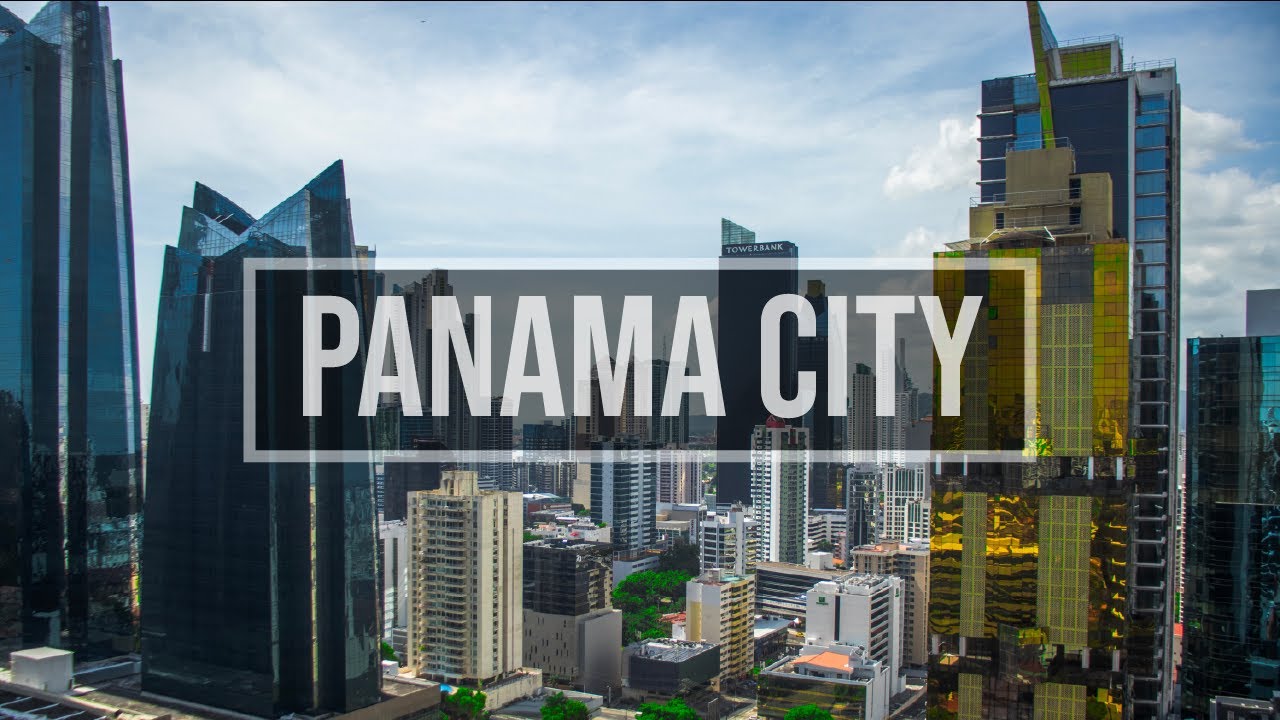This photograph captures a panoramic view of Panama City, prominently highlighted by the text "Panama City" in bold, block capital letters. The text is set within a slightly translucent white rectangle, allowing a glimpse of the vibrant cityscape beyond, while the letters remain fully opaque. The skyline is dominated by an array of high-rise buildings, showcasing a striking mix of black, blue, and gold mirrored facades. The high-rises stretch upwards, some disappearing out of the frame on both the left and right sides, while slightly shorter buildings fill the middle section.

The cityscape is set against a blue sky streaked with numerous white clouds, allowing only hints of azure to peek through. At the base of the towering structures, patches of lush green plants and trees add a touch of nature to the urban environment. The buildings display a variety of colors and materials, including white, tan, blue-gray, peach, and brown, with many featuring numerous windows. Among the structures, some appear to be parking garages or are possibly still under construction, adding to the dynamic, ever-evolving skyline of Panama City. The overall orientation of the image is rectangular, with the longer sides running horizontally, providing an expansive view of the city's architectural diversity.